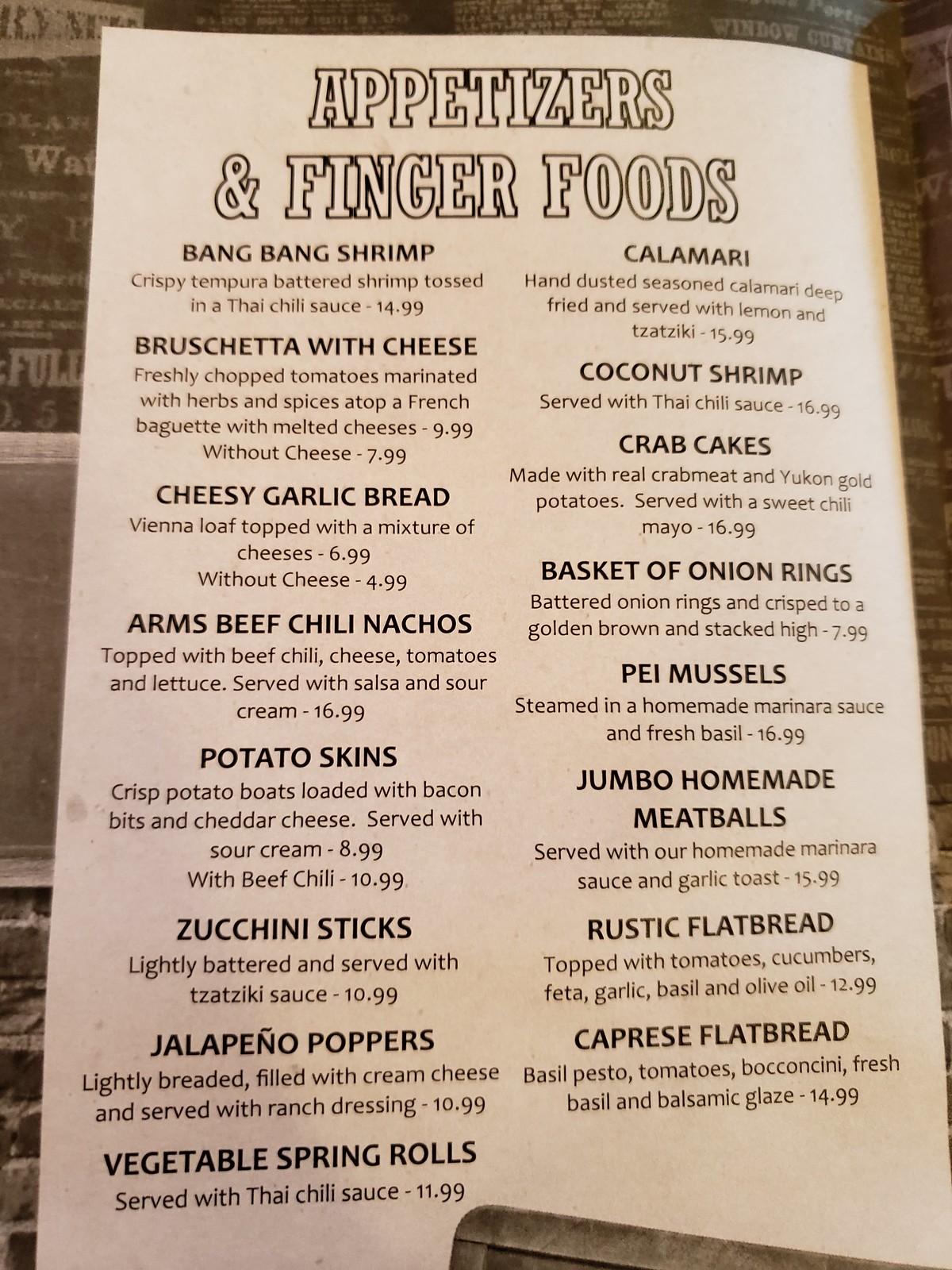This photograph captures a detailed view of a restaurant menu, specifically focusing on the "Appetizers and Finger Foods" section. The menu offers a variety of items including Bang Bang Shrimp, Bruschetta with Cheese, Cheesy Garlic Bread, Arm's Beef Chili Nachos, Potato Skins, Zucchini Sticks, Jalapeno Poppers, Vegetable Spring Rolls, Calamari, Coconut Shrimp, Crab Cakes, and a Basket of Onion Rings. Additionally, the selection features Hay Mussels, P.E.I. Mussels, Jumbo Handmade Meatballs, Rustic Flatbread, and Caprese Flatbread.

Highlighted prices on the menu include Calamari for $15.99, Rustic Flatbread for $12.99, Potato Skins with Sour Cream for $8.99 or with Beef Chili for $10.99, Jalapeno Poppers for $10.99, and Vegetable Spring Rolls for $11.99. 

In the background, there are glimpses of other publications and papers, with text visible, possibly indicating additional menu items or restaurant information.